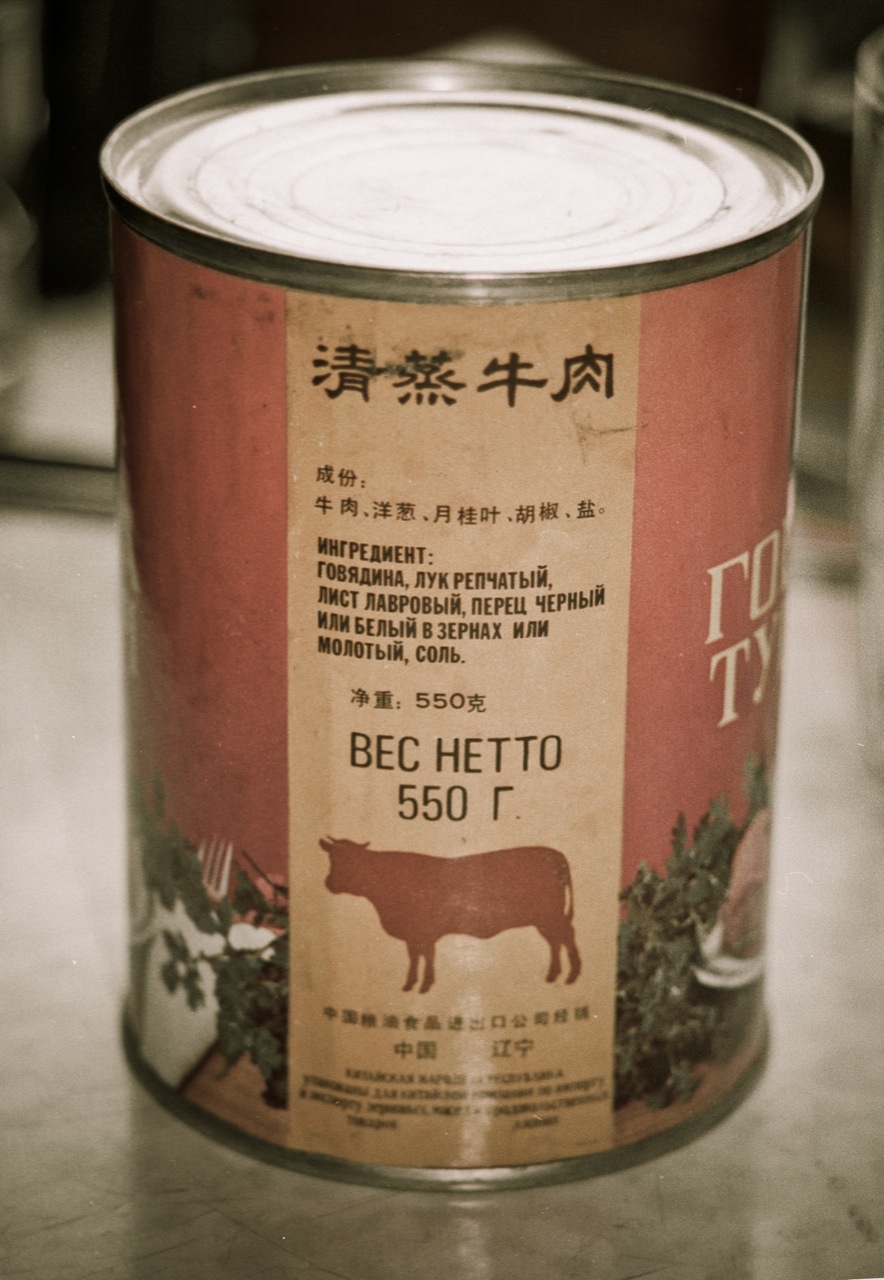The image showcases a can of food prominently marked with the number 550 multiple times. This old and smudged can features a combination of languages, including Chinese characters at the top and several lines of Cyrillic writing, likely Russian, below. The can itself is round and made of aluminum or tin, with a reddish label that transitions to a brown background in the center. This brown section is flanked by two red backgrounds. At the bottom of the brown background is a red silhouette of a cow, viewed in profile with two horns on the left side of its head. Below the red backgrounds, green leaves and a bowl with what appears to be meat are depicted. The top of the can is shiny aluminum, typical of a can designed to be opened with a can opener. The main part of the label also includes a detailed list of ingredients in Chinese and possibly other languages, although these details are hard to discern due to smudges and wear on the can's surface.